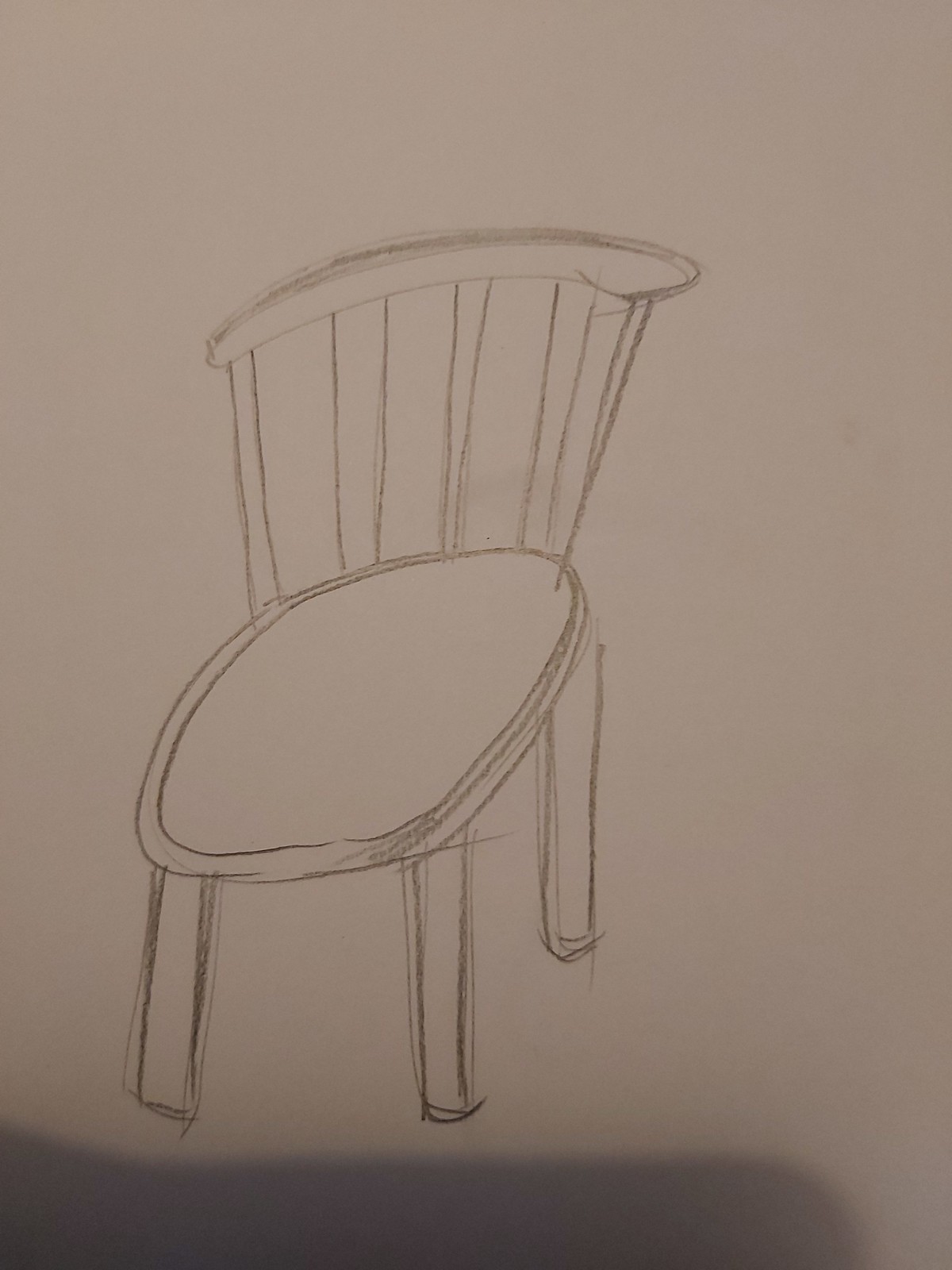A meticulously detailed pencil sketch graces a pristine white sheet of paper, capturing a classic wooden chair. The chair is oriented facing diagonally towards the bottom left corner of the page, providing a distinctive perspective that reveals only three of its legs. The chair's backrest features a rustic, fence-post style design with three or four vertical wooden slats, culminating in a gracefully rounded top. The expansive seat hints at a comfortable sitting experience, marked by a discernible outline that suggests the possibility of padding or cushioning. Despite its unfinished and somewhat rough nature, the sketch exudes a charming, early-stage artistic endeavor, showcasing the fundamental characteristics of a traditional wooden chair.